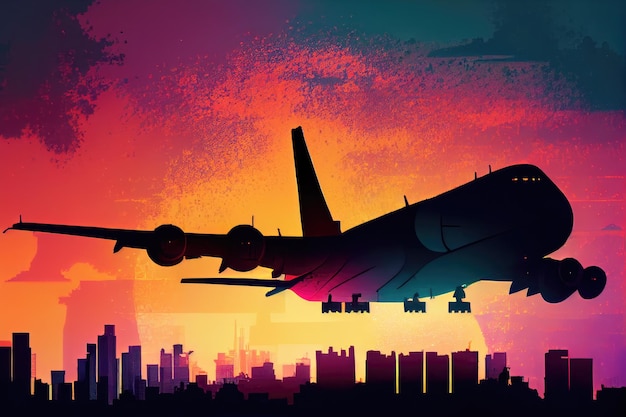The artwork is a painting depicting a large airplane front and center, its body ombre from gray and blue tones at the front to purplish and pink hues towards the tail, ending in a silhouetted black at the back and the engines. The sky forms a vibrant backdrop, transitioning from dark grayish or bluish tones in the upper corners to a dynamic blend of pink, fluorescent orange, and yellow as it reaches the lower half. The bottom of the image highlights a city silhouette with various tall skyscrapers, their shapes clearly defined but completely black against the colorful sky, resembling the effect of a setting sun. The airplane's cockpit is illuminated with narrow bands of light, and it features two engines on each wing.